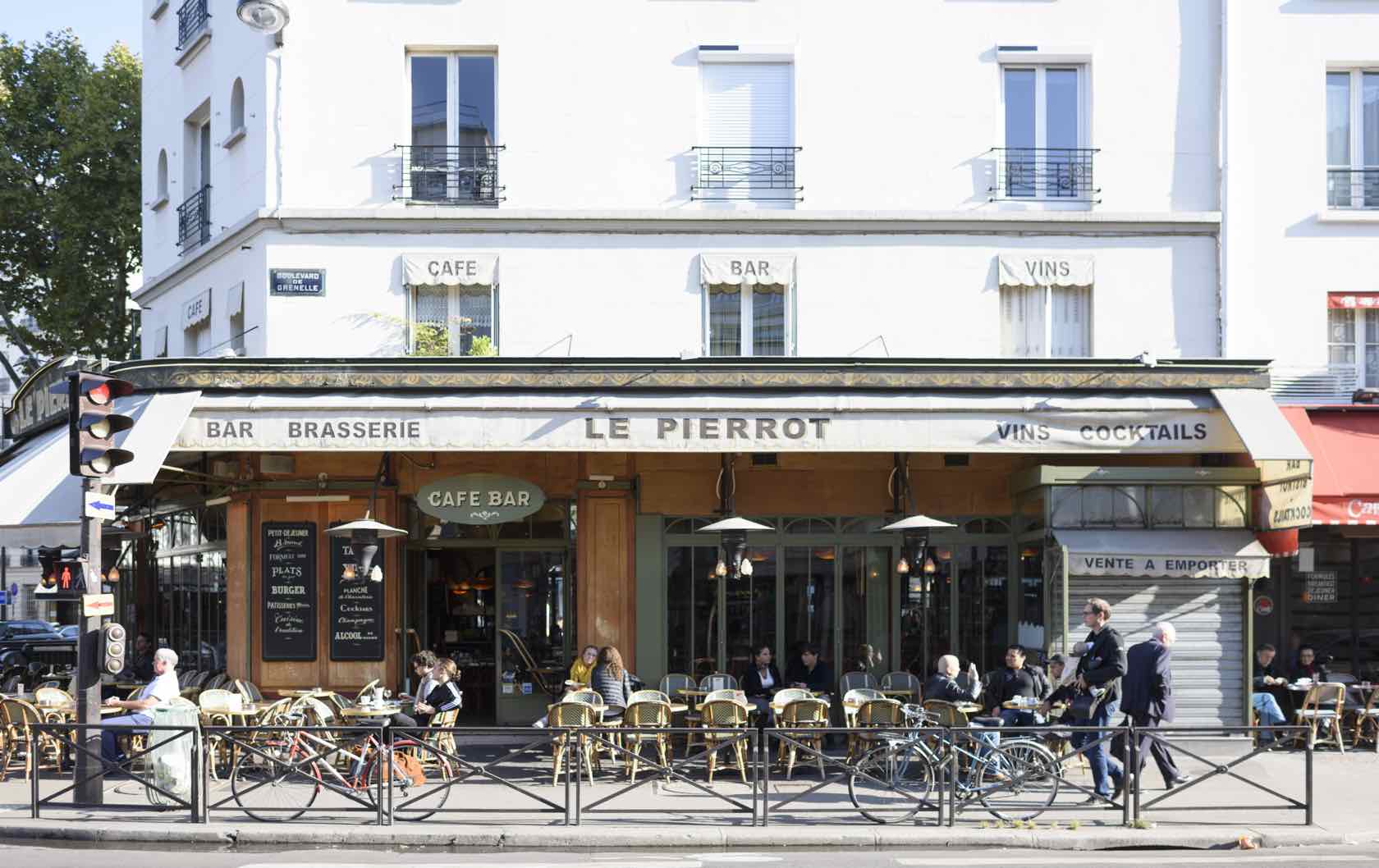This image depicts a bustling cafe bar in Paris, France. The establishment has a distinct, charming facade with a brown exterior and a white upper portion, possibly housing apartments or additional rooms. The cafe bar features an awning that reads "Le Pero" and underneath in bold lettering "Bar Brasserie à Vins Cocktails." The outdoor seating area is filled with numerous tables and chairs, many of which are occupied by patrons enjoying the pleasant weather. The cozy atmosphere is accentuated by bicycles parked alongside the building and various people walking by. Adjacent to the cafe, there's another restaurant with a red awning, also bustling with outdoor activity. The scene includes a traffic light in the vicinity, adding to the lively urban setting. Dark boards with white writing display the menu and specials, contributing to the inviting and vibrant ambiance of this quintessential Parisian locale.